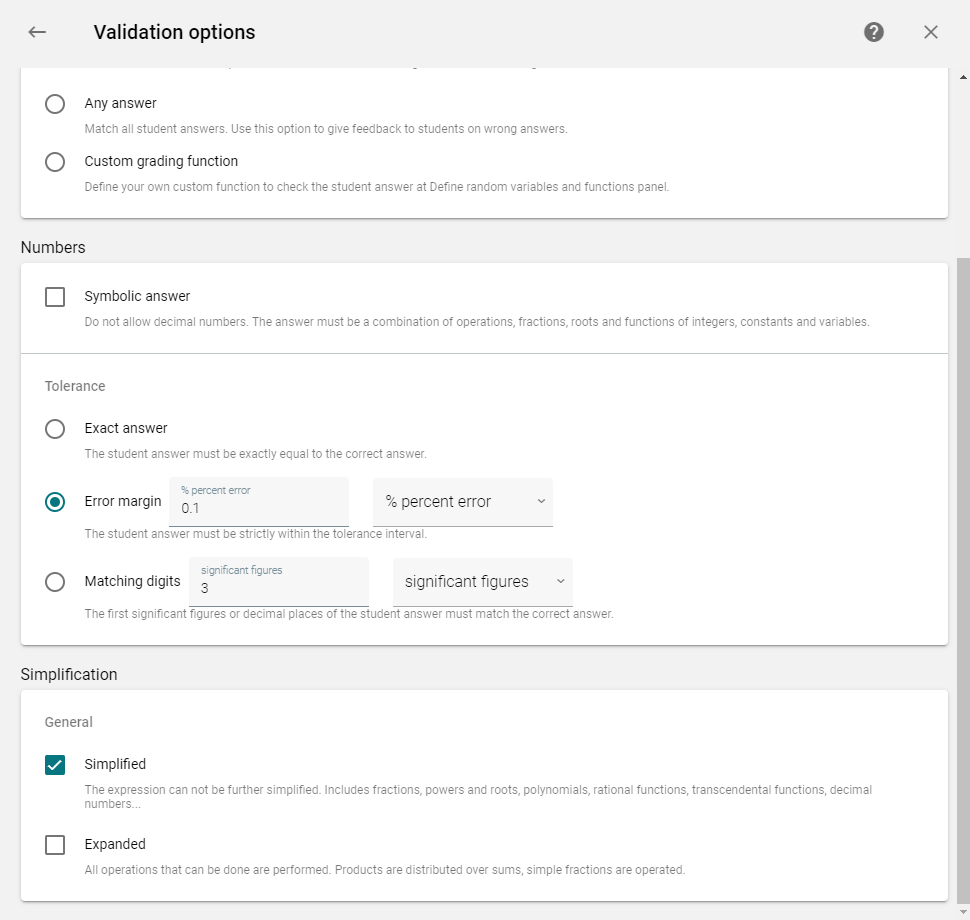The image shows a "Validation Options" panel on a website, set against a gray background. At the top left of the panel, the title "Validation Options" is displayed, accompanied by a left-pointing arrow. On the top right, there are two icons: a question mark for help and an 'X' for exiting the options screen.

Beneath the title is a white section containing two selectable options: "Any Answer" and "Custom Grading Function". Further down, the category "Numbers" is labeled in small black font, followed by a large white area. At the top of this section, "Symbolic Answer" is indicated, with an unchecked checkbox to its left. Below this, under the subcategory "Tolerance," are the options for "Exact Answer," "Error Margin," and "Matching Digits." The "Error Margin" option is selected, with two adjacent fields specifying a 0.1% error margin and the unit "Percent" being selected.

At the bottom of the panel, the "Simplification" section is detailed, featuring another white box. In this section, "General" is displayed at the top left, followed by choices for "Simplified" and "Expanded." Here, "Simplified" is selected.